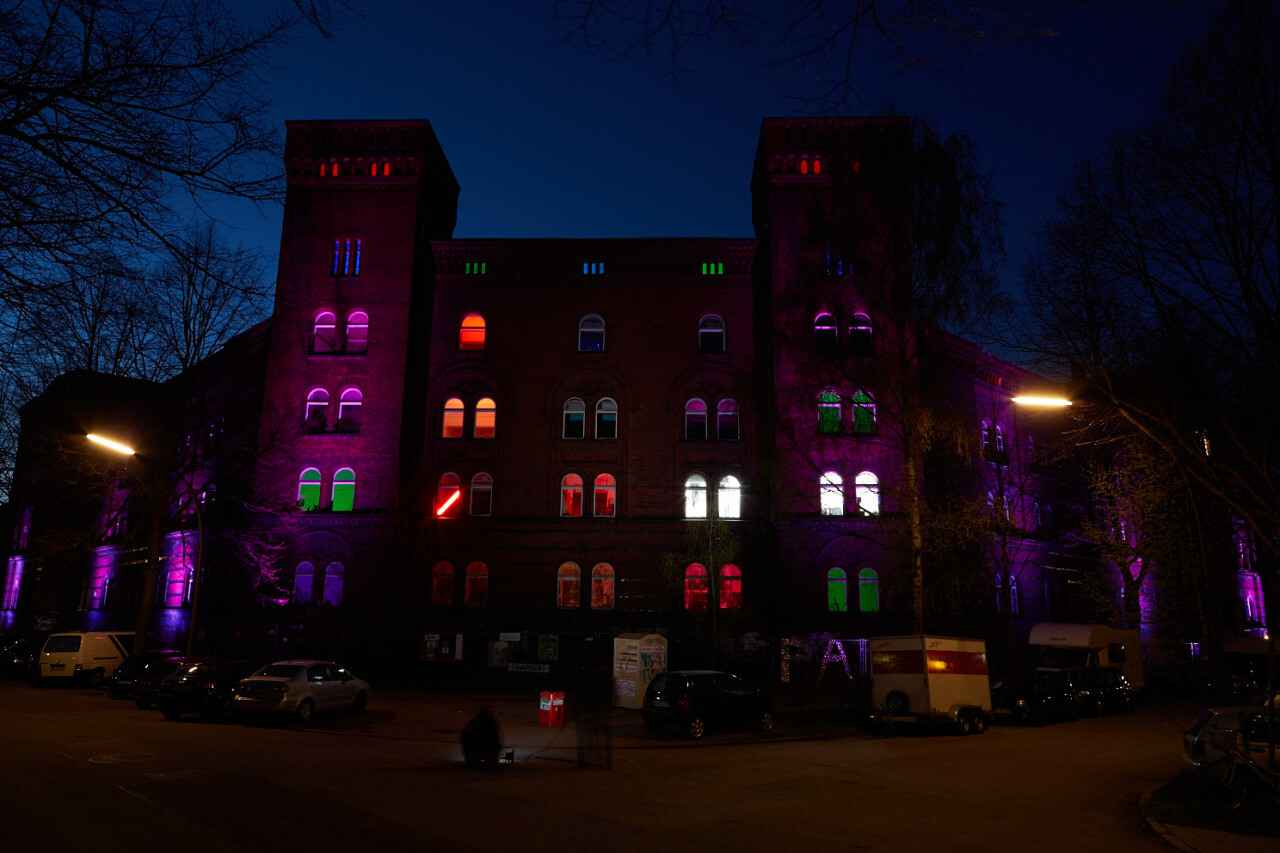This color photograph depicts a large, multi-story brick building at night, framed by trees on either side against a dark blue night sky. The building is five stories tall at its main sections, with two tower sections at each corner that extend to six stories, and a seventh story for the towers. Many windows are illuminated in various colors, including red, blue, green, orange, white, and pink, significantly adding to the visual appeal. The bottom levels feature arched windows, with smaller windows at the top levels. The sides of the building are lit with blue lights, and the towers have additional red-lit windows at their pinnacle. 

In the foreground, a street is visible with several parked cars, including some trailers and a vehicle pulling a camper. A man is crouched on the ground, illuminated by a nearby light. A porta-potty can also be seen among the vehicles, adding to the street-level details. The overall scene portrays a vibrant and lively atmosphere under the night sky.